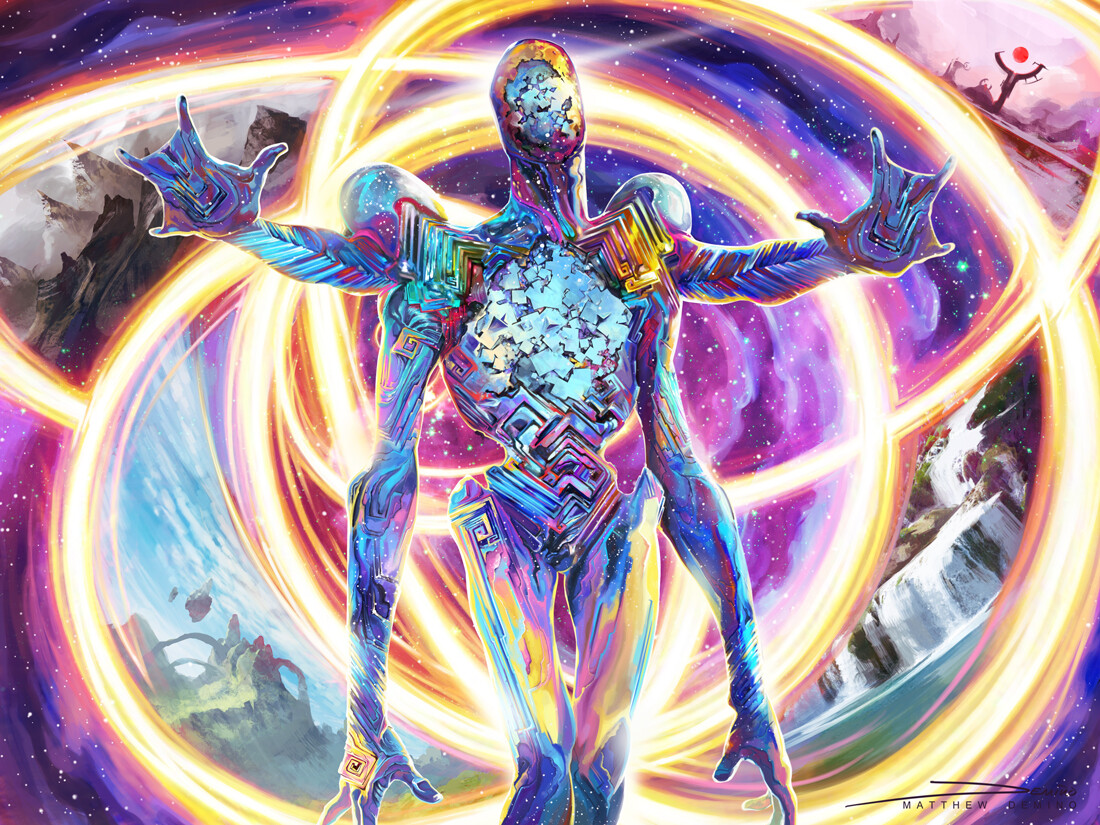The image depicts a fantastical creature with a translucent body, intricately composed of interwoven lines and geometric shapes in a mesmerizing kaleidoscope of colors, predominantly gold, silver, purple, and blue, with hints of other hues. This ethereal being has the head and neck of a human but possesses four arms, each hand featuring only four fingers, as well as two legs. Notably, the creature lacks facial features such as eyes, a nose, or ears. The background is equally captivating, featuring a complex array of intersecting and interlocking circles colored in a spectrum of gold, yellow, purple, pink, brown, and gray. Within the lower left and right sections of these circles, detailed landscapes of rocks and waterfalls can be seen, adding depth and mystique to the scene.